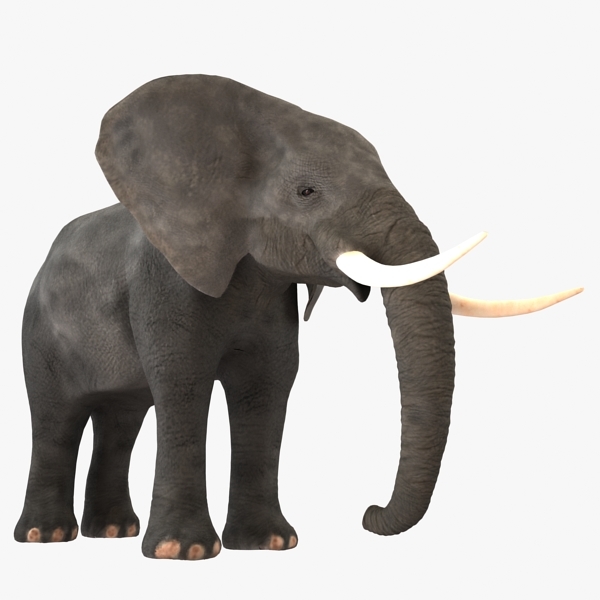The image features a digitally rendered elephant set against a completely white background. The elephant is oriented to the right and slightly angled, with its front end closer to the viewer than its rear. This detailed rendering showcases the elephant's distinctive features: it has large, leathery gray ears, a long trunk that bends slightly inwards, and striking white tusks that protrude from either side of its trunk. Its skin appears dry and cracked, adding a tactile, smoky light gray texture to its form. The elephant's visible right eye is black, and it has small white nails or toes with a slight pinkish hue at the ends of its feet. The overall impression is of a young elephant, though its exact age is uncertain. The composition emphasizes the natural, intricate detailing of the elephant's anatomy against the stark simplicity of the background.